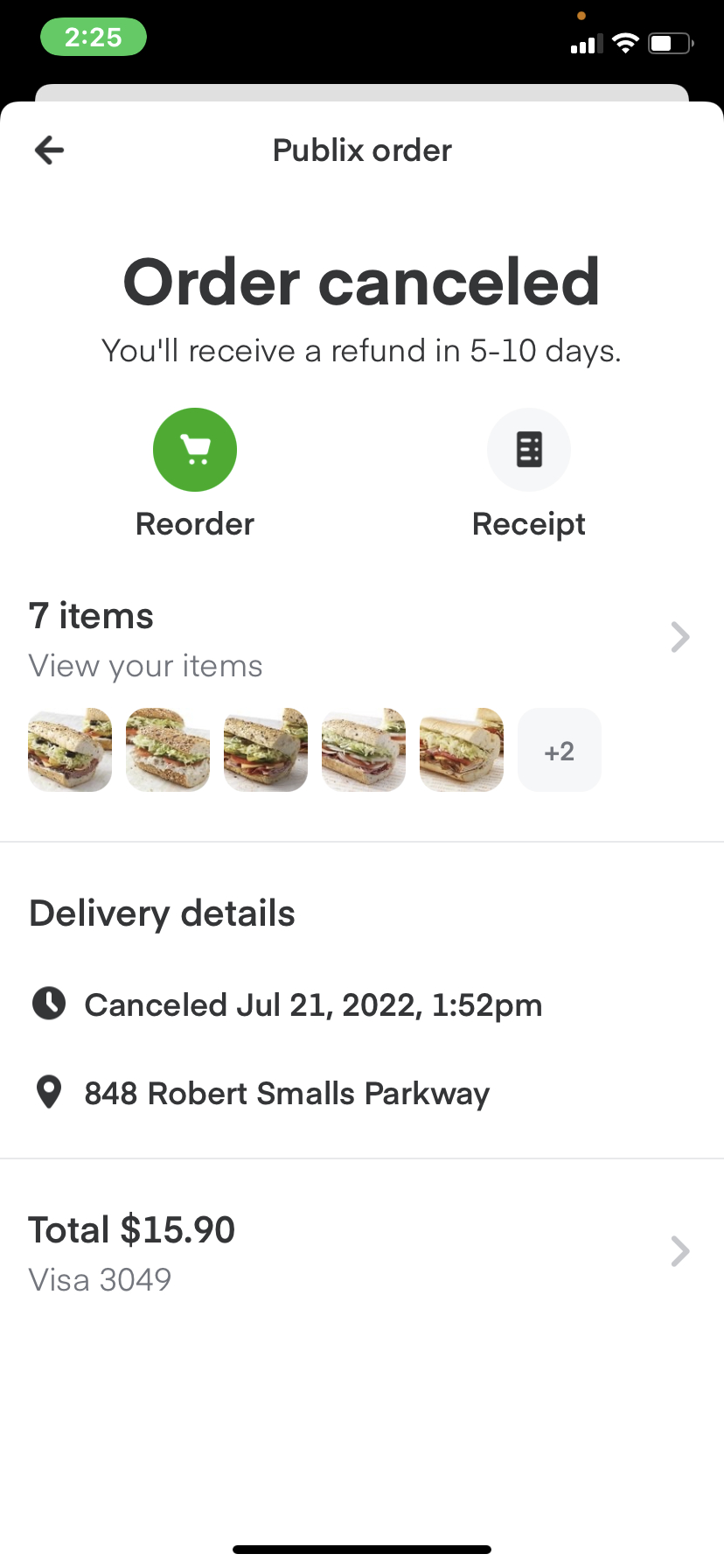The image appears to be a screenshot from a smartphone. At the top of the screen, there's a status bar with various indicators: a green oval encloses the time, which reads "2:25" in white text, alongside signal strength bars, a Wi-Fi icon, and a battery icon, all set against a black background with white text.

Below the status bar, the main content of the page is displayed on a white background. At the top-left corner, there's a back button followed by the text "Publix Order" in bold. Centered on the page is a prominent notification stating "Order Cancelled" in large text, with a message below indicating that a refund will be processed within five to ten days.

Further down, there are two interactive buttons: a green circle with a shopping cart icon labeled "Reorder," and a light gray circle with a black list icon labeled "Receipt." The text "7 Items" is shown with a note in light gray beneath it saying "View Your Items."

The image section includes five pictures of what appear to be sub sandwiches, followed by a gray box with the text "+2," suggesting there are more items. A gray arrow to the right indicates that clicking it would likely reveal further order details.

Next, under the heading "Delivery Details," the order status reads "Cancelled," with a timestamp: "July 21st, 2022, 1:52 PM," and the delivery address: "848 Robert Smalls Parkway." A separator line designates the order's total cost as "$15.90," with the payment method noted as "Visa 3049." Another right-pointing gray arrow suggests additional receipt details are available if clicked.

At the bottom of the screen, a gray bar—that potentially acts as a control center or menu access point for the phone—is partially visible, indicating it might be swiped up for more options.